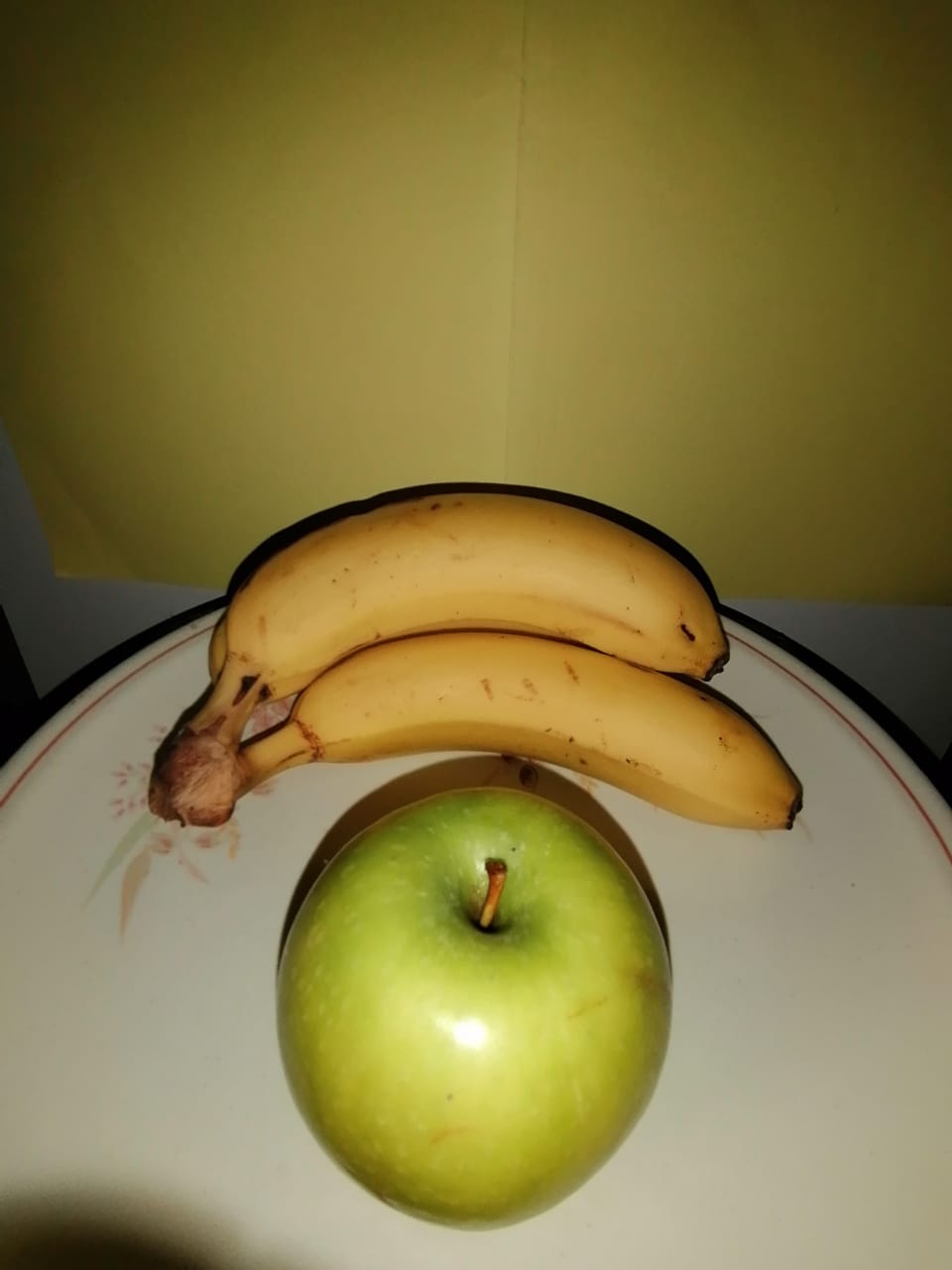A meticulously arranged composition features a white plate with a delicate gold trim approximately a quarter inch from its rim. The plate is positioned against a stark white background, with a seam indicating that the yellow wall behind it is actually comprised of two yellow pieces of paper taped together. Dominating the center of the plate is a vibrant green apple, complete with its stem intact. Perched above the apple are two slightly overripe bananas still attached at the stem, forming a protective arch over the apple. The bananas' stems rest on a subtle, peach-colored and light green print that extends partially under them, though the exact design remains obscured. Despite their close proximity, the apple and bananas do not touch; a clear shadow cast by the bananas falls between them, adding depth to the scene. An additional shadow appears in the lower left-hand corner of the plate, possibly belonging to the person who took the photograph. The careful placement of the fruits and the interplay of shadows make for an aesthetically pleasing and thoughtfully composed image.